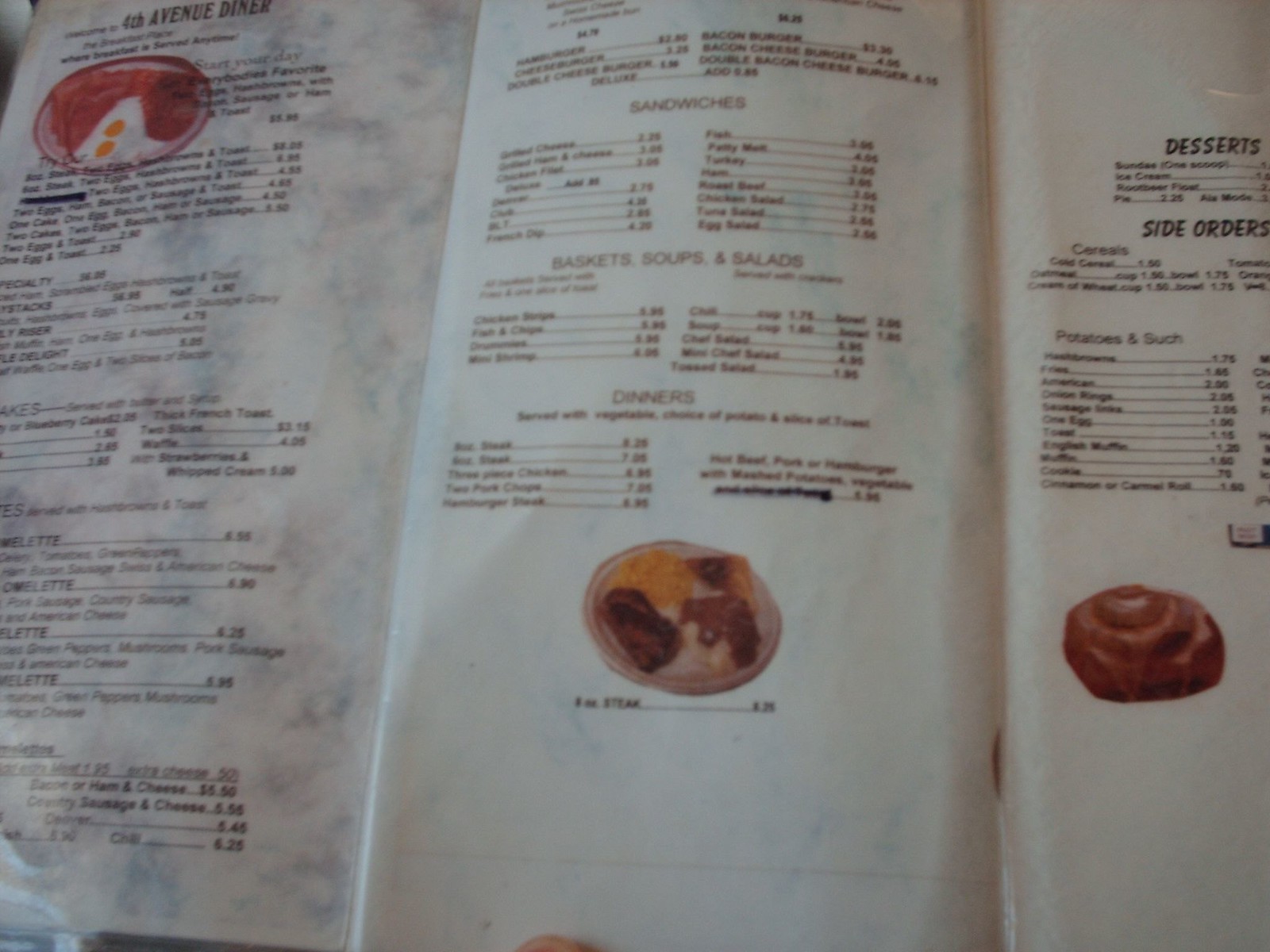The photograph captures a fully open rectangular menu from 4th Avenue Diner, divided into three distinct columns. 

The first column features a marbled background with light blue swirls resembling clouds, set against a cream base. The top left corner displays the diner’s name, "4th Avenue Diner," alongside an image of two fried eggs encircled by a brown arc, implying a hearty breakfast. The text announces, "Start Your Day, Everybody's Favorites," listing options like steak, various cakes, and eggs. Further down, headings such as "Specialty Stacks" and "Pancakes" introduce the breakfast section, which includes multiple types of omelets. The bottom of this column highlights affordable selections like ham and cheese, and sausage and cheese, along with their prices.

The second and third columns utilize plain cream backgrounds. The second column begins with "Sandwiches" at the top, proceeding to categories like "Baskets," "Soups and Salads," and "Dinners." An image near the column’s bottom likely features mashed potatoes with gravy, steak, and corn, although the fourth item is unclear.

Leading into the third column, a staple appears at the bottom right, with an image of a Danish positioned above it. The third column starts with "Desserts," offering sundae options and various ice creams. Further categories include "Side Orders," listing options such as cereals (cold cereal, oatmeal), and a variety of potatoes and such items like hash browns and french fries. Additional items include American favorites, onion rings, sausage, and single eggs.

This menu provides a thorough view of the diner's offerings, highlighted by rich visual details and easily navigable sections for a variety of meals and snacks.